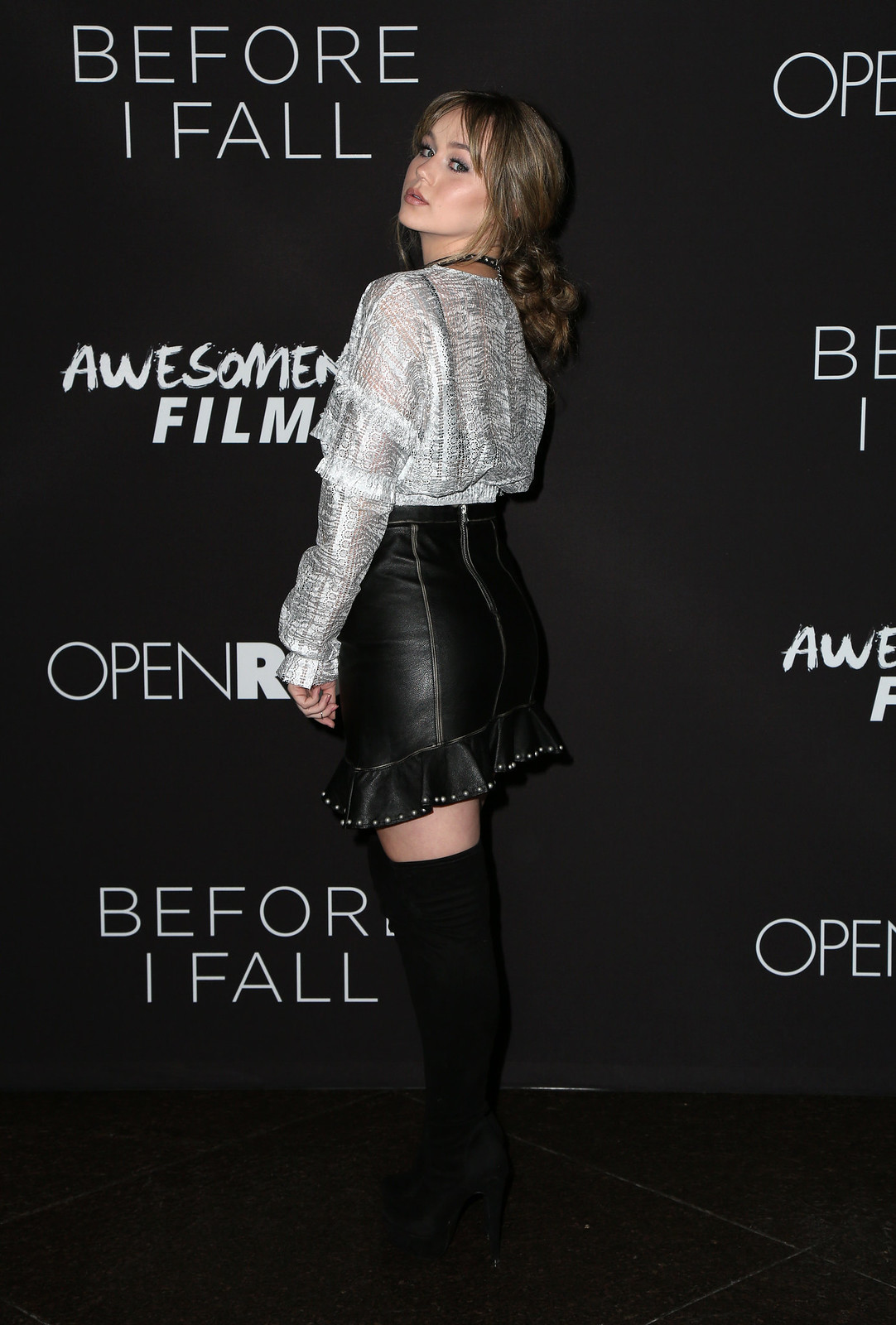In this striking color photograph, a young Caucasian woman takes center stage, posing confidently against an all-black background. Her brown hair, styled into a loose yet curly ponytail, accentuates her poised demeanor. She is dressed in a chic ensemble featuring a white long-sleeve top, a form-fitting leather skirt, long black socks, and black shoes. A black necklace adds a touch of elegance to her look. Standing with her back slightly arched, her body faces the 10 o'clock position while her head is turned over her left shoulder, her eyes directed towards the camera. The black-tiled floor beneath her complements the dark wall behind, which is adorned with multiple phrases in white text. Dominant among them are "Before I Fall," and "Awesome Film," appearing prominently on the left side and repeating at the bottom. The text "Open R" is partially visible in some places, contributing to the layered typography on the wall. The image captures both her stylish outfit and the evocative backdrop, creating a compelling visual narrative.